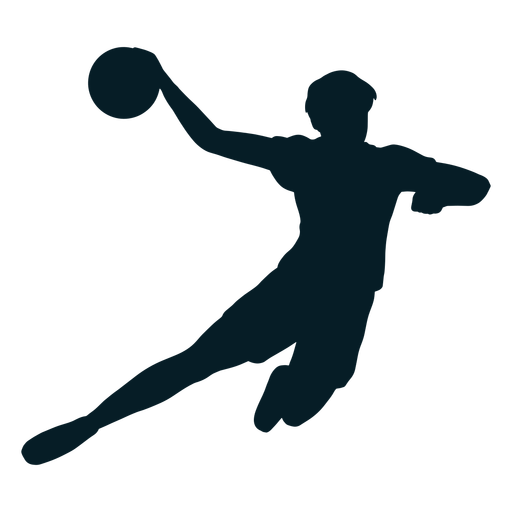The image showcases a black silhouette of a man, possibly a basketball player, set against a white background. He is depicted mid-jump, with his right hand outstretched to the west, holding a basketball high in the air. His left hand is balled into a fist and positioned in front of him, adding dynamic motion to the scene. His right leg is extended straight out at a 45-degree angle, while his left leg is bent at the knee, contributing to an impression of leaping. The figure features short hair and appears to be wearing a t-shirt, shorts, and sneakers, although the silhouette offers no detailed facial features or clothing specifics. The image evokes a sense of athleticism and could be reminiscent of the famous Nike "Jumpman" logo, though it is distinct and not an exact replica.